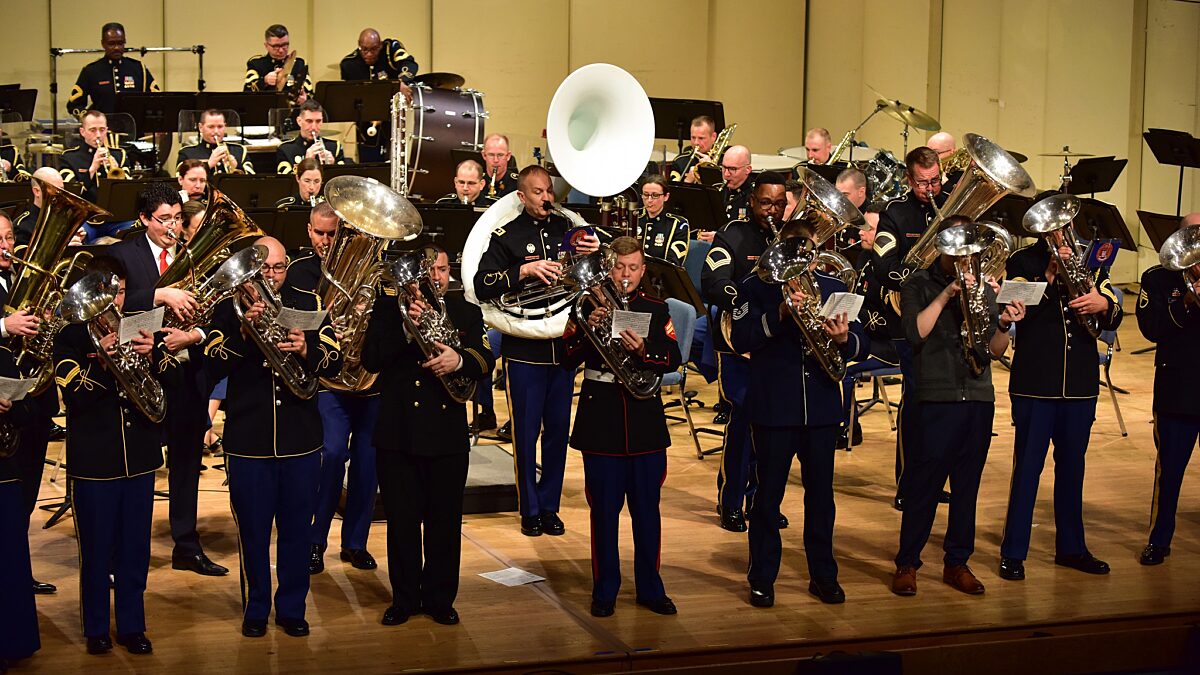The photograph depicts a United States Marines military band performing on a shiny, light brown wooden stage. The stage is backed by a plain cream-colored wall, segmented by vertical lines that give the appearance of slats. The band consists of about 30 members, all clad in their formal dress uniforms, distinguished by blue coats with red trim and black shoes. Each band member is standing, with few, if any, seated behind and obscured by the front row. The musicians are predominantly playing wind instruments, including saxophones, trumpets, trombones, and a very large white tuba held by a central figure. Towards the back, a few members are playing drums and cymbals. Some band members appear to be reading from sheet music placed on black stands, adding to the disciplined and organized scene.